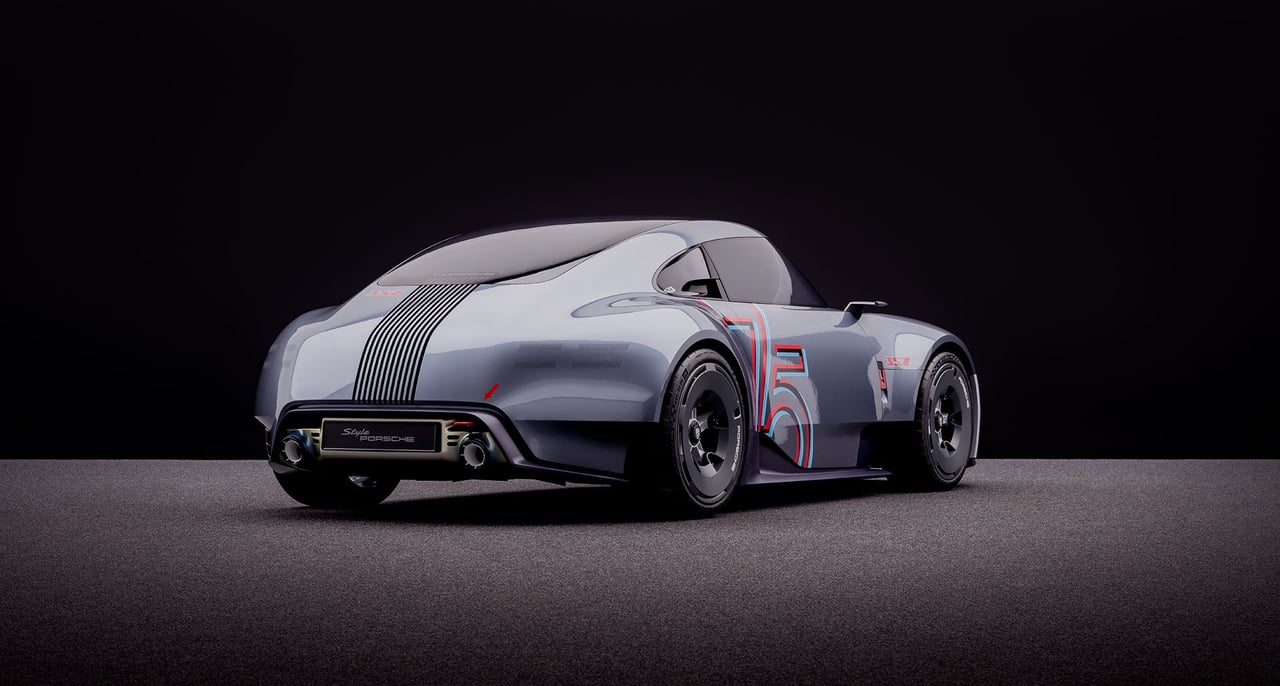The image showcases a dramatically lit scene with a bluish-gray race car parked on a gray surface, contrasting starkly against a completely black background. The car, which has black wheels and solid black tinted windows, exudes an aura of speed and performance. The vehicle, reminiscent of a vintage hot rod with curvy, rounded lines akin to a Bugatti, features a distinct number 75 embossed on its side. It also sports squiggly red lines on the right side door and dual exhausts at the back. Despite the car facing away from the photographer, its new, reflective paint and minimalistic frame design are clearly visible. Although there is an odd dent in the back, this might contribute to its aerodynamic form. The surface it rests on, described alternately as a gray carpet or asphalt, enhances the visual impact of the black rims and tires, making them look like a single unit.